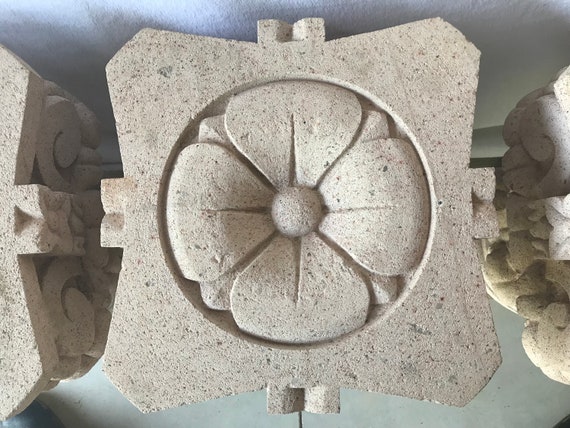The photograph showcases a collection of stone sconces arranged side by side in what appears to be a warehouse setting. These sizable sconces, approximately 16 by 16 inches, are intricately carved with a floral design. Each sconce features a four-petaled flower with narrow petals that flare out, resembling a beaver's tail. The gently curving petals converge toward a round central piece that matches the flower’s tan hue, interspersed with black spots. The sconces exhibit a slightly imperfect, not entirely square form, with a shape that's both pointy and curvy at the edges. The background consists of a whitish-blue surface, possibly a marble wall or tabletop, further highlighting the light tan and beige tones of the stone sconces.